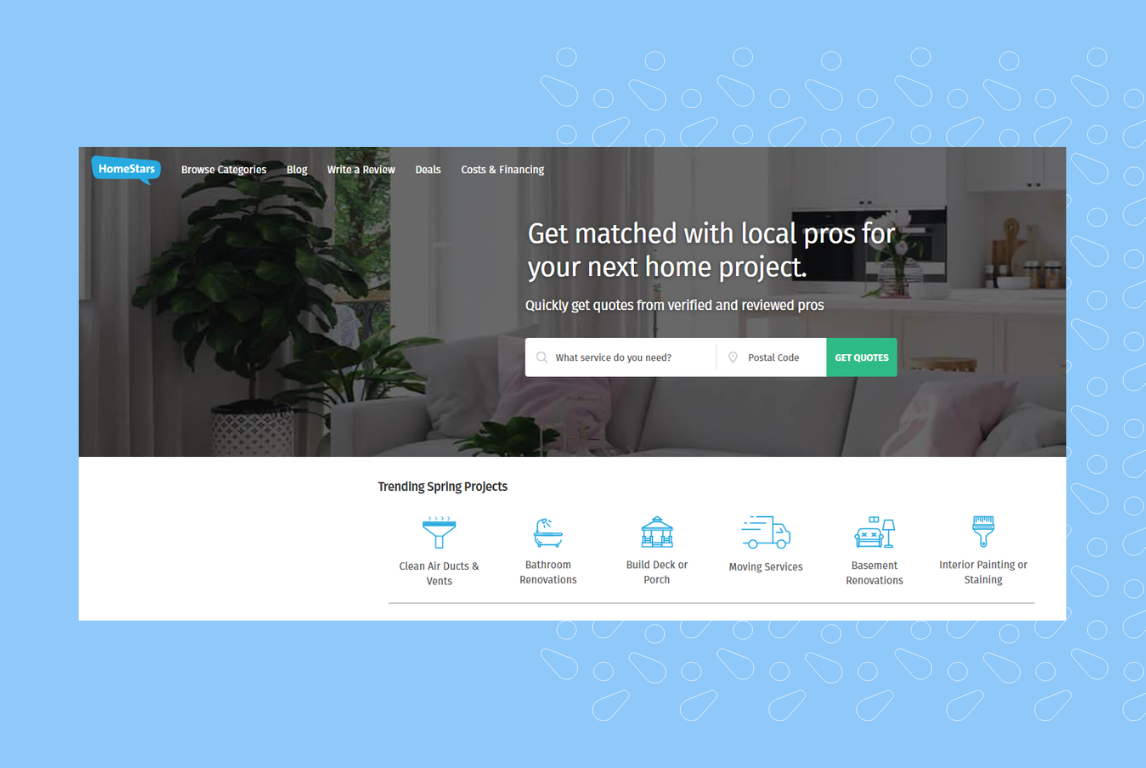The image showcases a serene home improvement website interface with a light blue background. The header features white text categories: "Home," "Stars," "Browse Categories" (twice), "Blog," "Writer Review," "Deals," and "Cost and Financing." 

Prominently displayed is a picturesque photograph of an elegant home interior, highlighting Venetian blinds, a potted plant, and a pristine white couch adorned with white and light pink pillows. Visible in the background is a modern kitchen with a cohesive white color scheme. Overlaying the image, a headline reads, "Get matched with local pros for your next home project. Quickly get quotes from verified and reviewed pros."

Beneath the headline, a search bar allows users to enter their postal code, with a green "Get Quotes" button in white text. Additionally, the site promotes "Trending Spring Projects" with blue-tinted sections listing services such as clean air ducts and vents, bathroom renovations, build dock or porch, moving services, basement renovations, and interior painting or staining. The clean and organized layout aims to connect users with professional home improvement services efficiently.